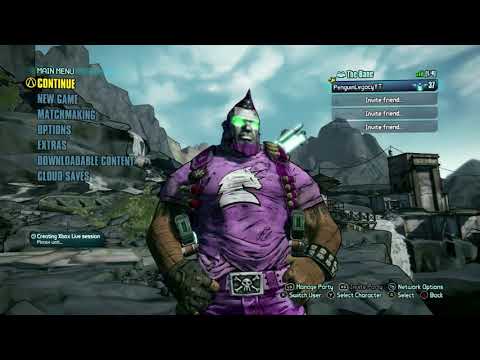This image is a detailed screenshot from one of the Borderlands video games. At the center stands a brawny, dark-skinned character with immense, muscular arms, which are almost as thick as half the width of his body. His distinct features include a blue mohawk, a blue beard, and shining yellow glasses. He wears a dark purple T-shirt emblazoned with a white unicorn and dark purple pants with a purple belt that features a skull and crossbones emblem. Additionally, he sports a glove with cut-out fingers on his right hand and a large, riveted black bracelet on his left wrist. 

The screenshot showcases an alien sci-fantasy setting with a backdrop of gray rocky mountains, a blue sky, and a small waterfall to the right, crowned by a building atop it. Interface elements are visible throughout the image, albeit mostly illegible due to their small size. On the left, a dark bluish-gray overlaid menu displays 'Main Menu' in bold, followed by 'Continue' in bright yellow, and subsequent options including 'New Game', 'Matchmaking', 'Options', 'Extras', 'Downloadable Content', and 'Cloud Saves'. Another floating menu to the right features options for inviting friends into the game.